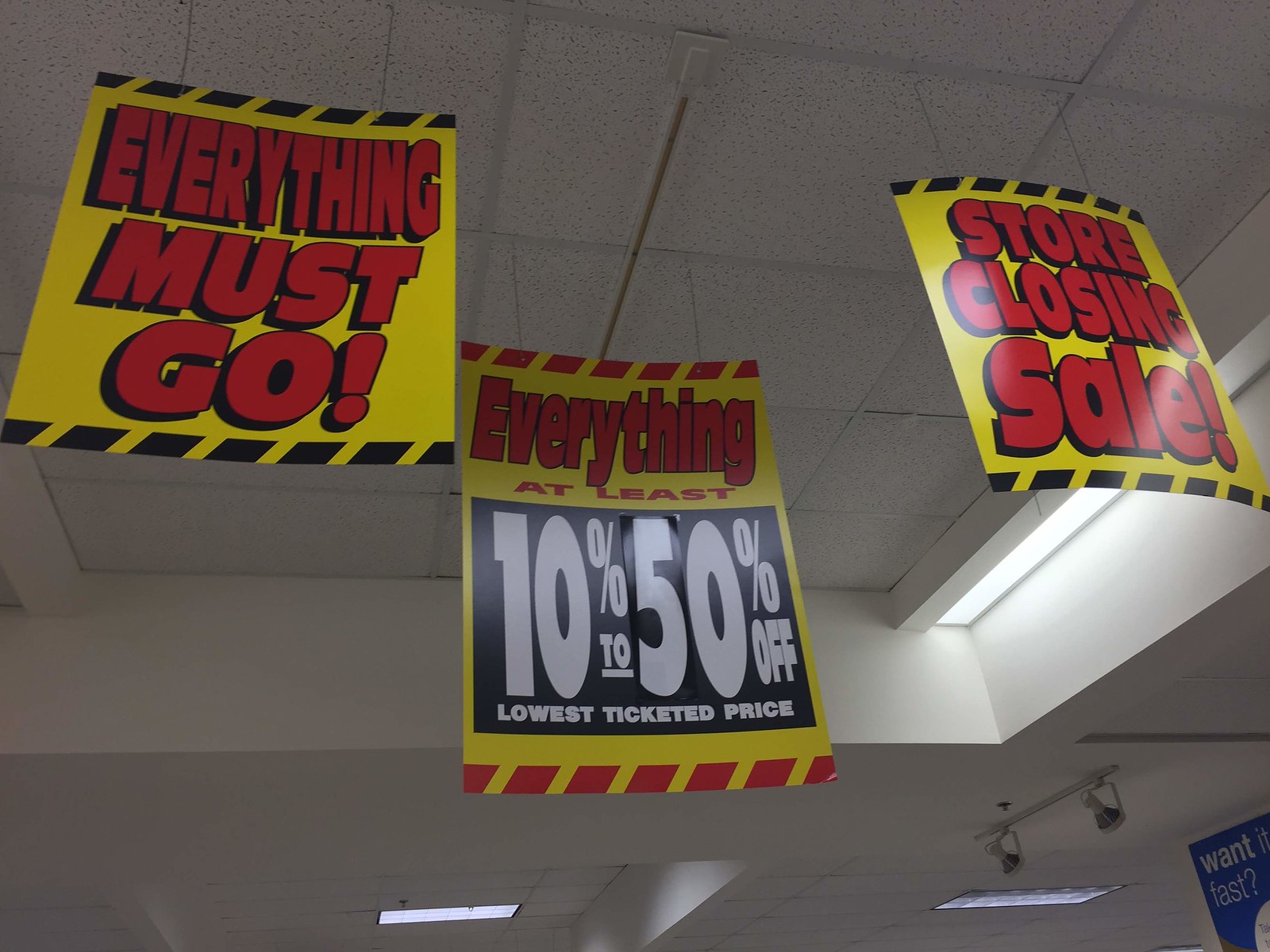This photograph captures the interior of a store, with the camera angled upwards toward the ceiling. The ceiling itself is composed of white panels, and is visibly populated with overhead incandescent lights, emitting a white glow, which are commonly found in retail establishments.

Prominently featured in the image are three yellow signs that hang from the ceiling. These signs, resembling flat banners made of a plastic or paper-like material, are filled with bold red text proclaiming, “Everything Must Go,” “Everything At Least 10-15% Off,” and “Lowest Ticketed Price.” Notably, the “10-15% Off, Lowest Ticketed Price” portion stands out with white text set against a black background. These signs indicate a store closing sale, emphasizing the urgency and discounted prices.

In the bottom right-hand corner of the photograph, a partially visible blue sign displays the text “Wanted? Vast?” Though the sign is clipped and not entirely legible, it adds to the cluttered, liquidation atmosphere of the image.

Additionally, the scene includes various functional elements of the building’s infrastructure, such as pipes and potential water lines extending downward from the ceiling. This detail, along with additional floodlights near the blue sign, contributes to the industrial aesthetic of the store's interior.